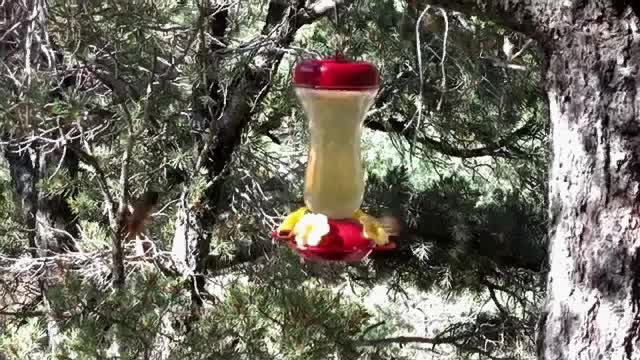This detailed image captures a hummingbird feeder hanging from the branch of a large pine tree, its rough, scraggly bark in shades of silver and gray visible on the right-hand side. The pine tree, along with numerous others in the background, contributes to the dense, heavily wooded forest setting. The hummingbird feeder has a distinctive vase-type shape with a flared-out top and is made primarily of plastic. It features a bright red round lid and a red dish at the bottom to attract hummingbirds. Four small yellow plastic flowers encircle the base, each acting as a feeding port. The feeder’s central cylinder, constructed from clear plastic or glass, contains a cloudy, slightly yellow liquid, indicative of hummingbird food. This scene, with its interplay of light and shadow on the tree trunks and branches, conveys the tranquility and fullness of the forest environment.